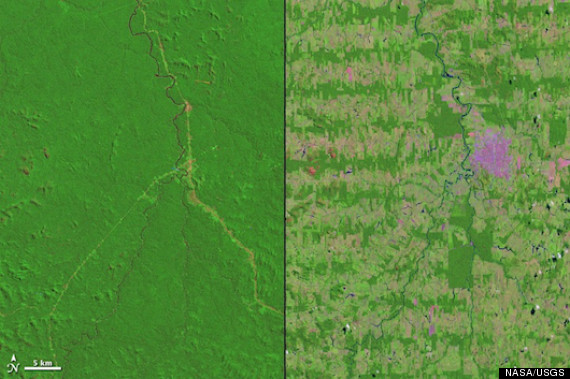The image features a digitally constructed, side-by-side topographical map predominantly rendered in green hues. In the lower right corner, a black rectangle with the white text "NASA USGS" marks the origin of the images, hinting at satellite involvement. The lower left corner showcases a compass symbol with an "N" for north and an upward-facing triangle, alongside a white line scale indicating "5 km."

The left section of the map is almost entirely green, displaying a river flowing from the top, slightly rightward as it progresses downward, and then forking into three branches. A red or orange line runs vertically adjacent to the river, shifts direction diagonally, and continues vertically again, with an offshoot line branching out. The texture in this section evokes the rough, raised surfaces one might observe on heavily textured art or walls, with a striking gold crack resembling lightning.

In contrast, the right section exhibits more striated green areas interspersed with clusters of pink, along with some brown tones. A vertical blue crack cuts through this part of the map, exposing a mauve circle with rough edges. The green areas here are less uniform, and the river is flanked by more varied hues, including purple clusters in the middle right. This dual-filtering effect accentuates topographical differences and possibly highlights geological or vegetative variations in the landscape.